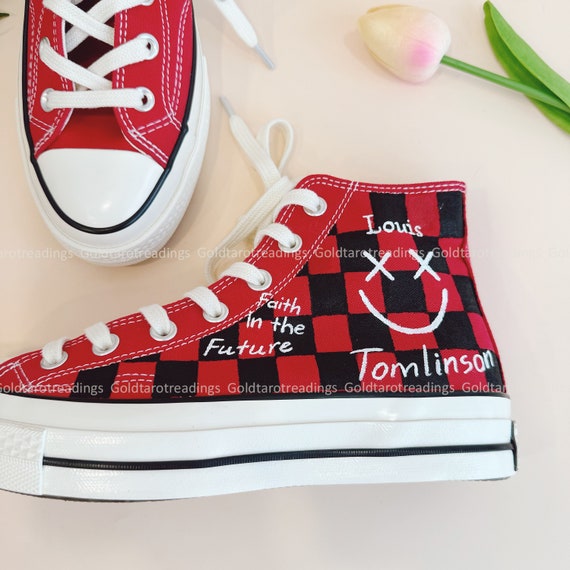This photograph, taken indoors, showcases a pair of high-top sneakers with a red and black checkered pattern. The style is reminiscent of basketball sneakers and appears to be Converse, given their distinctive design. Both sneakers have white soles, white toe caps, and white laces. One shoe is positioned on its side, displaying detailed handwriting elements, while the other stands upright in the upper left corner, viewed from above.

On the side of the shoe lying down, the text "Lewis" is written near the heel, accompanied by a smiley face with X's for eyes, and the name "Tomlinson" is placed below it. Additionally, the phrase "Faith in the Future" is inscribed to the left of these details. The setting includes a pale peach-hued white tabletop and subtle watermarks in light gray that read "Gold Tarot Readings," repeating across the image. A delicate tulip, showcasing pale pink and white petals with a green stem and leaf, is positioned in the top right corner.